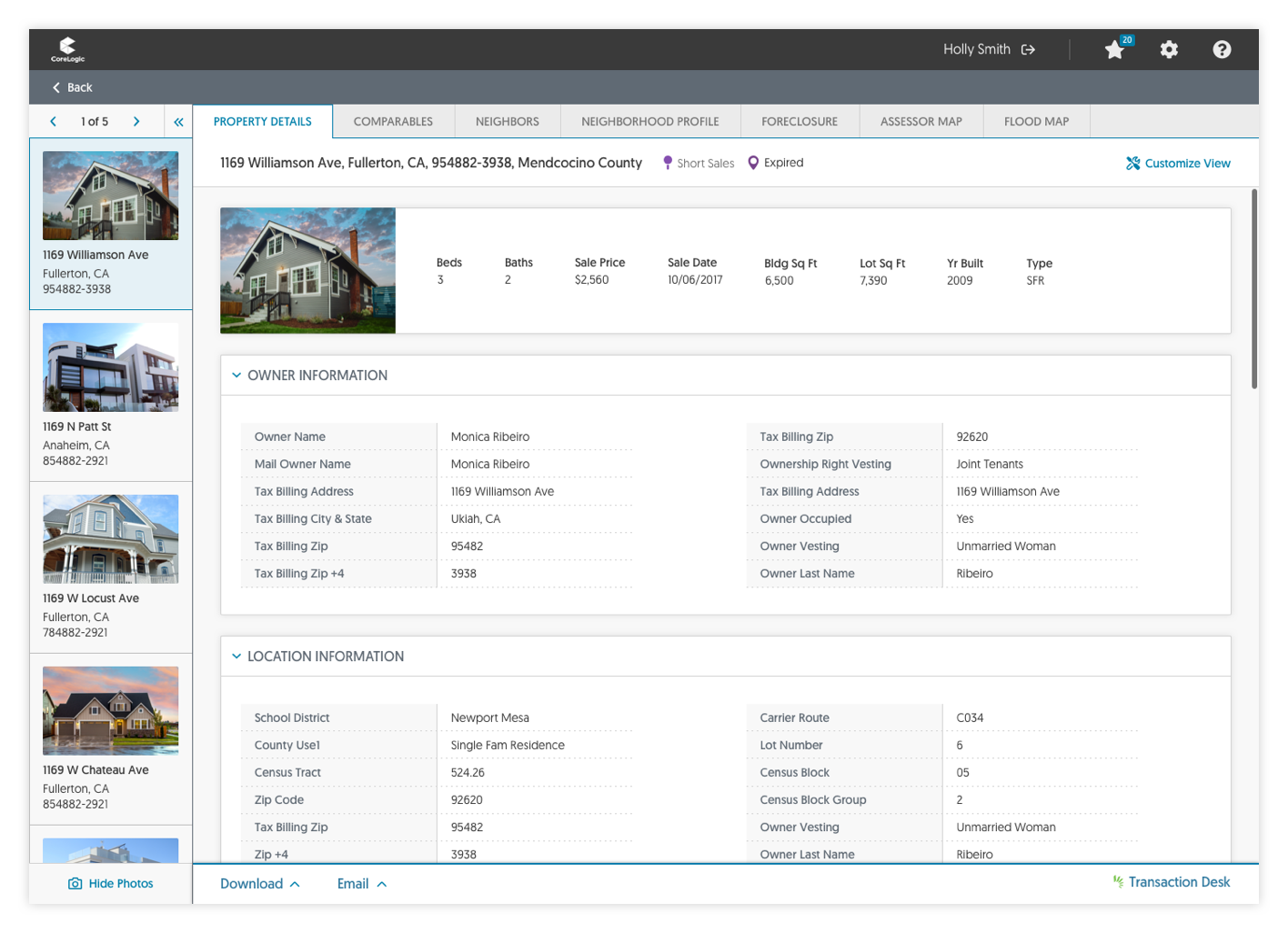The image depicts a realtor website interface, presumably named "ConLogic," where the user is logged in as Holly Smith. At the top of the webpage, the ConLogic logo or title is somewhat unclear. Along the left-hand side, there's a vertical column showcasing photos of homes alongside their addresses, confirming the site's purpose for real estate listings. Visible in the column are four full-sized property images along with a fifth partially visible image at the bottom. When a property image is clicked, a detailed page opens to the right of the screen, providing comprehensive information about the selected home. The highlighted property is located at 1169 Williamson Avenue in Fullerton, California. This detail page includes essential data such as the number of bedrooms and bathrooms, the sale price, the sale date, and the total square footage of the property. Additionally, there is an "Owner Information" section followed by a "Location Information" section, providing further insights about the listing.